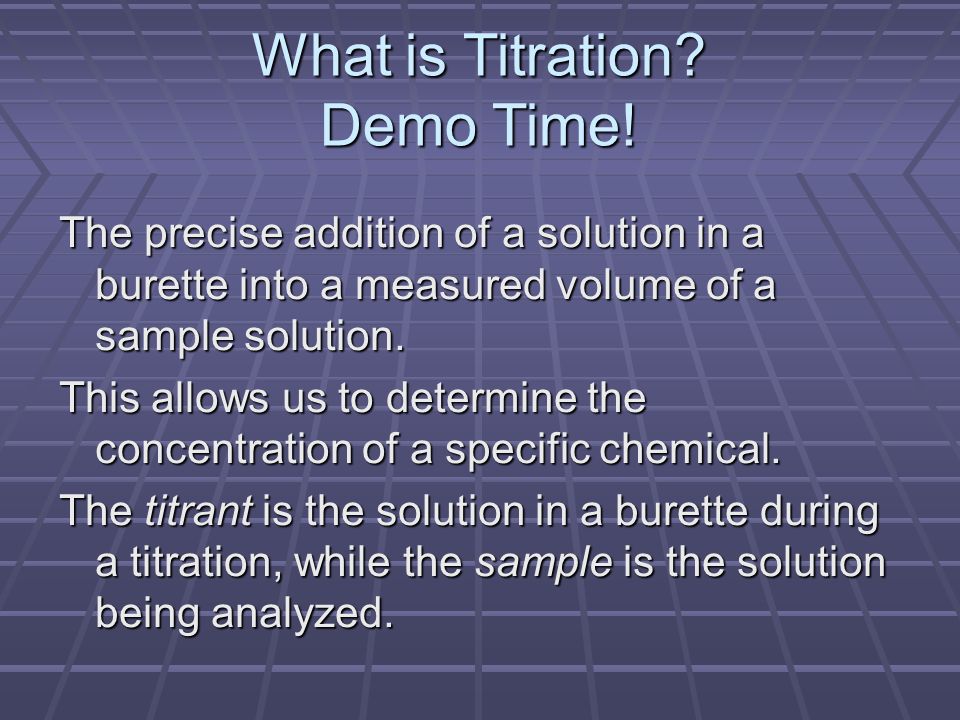The image displays a PowerPoint presentation slide with a detailed explanation of titration. The background features a purple design with various shades of purple lines running through it. The title at the top of the slide is in large, white (or possibly light blue) text that reads, "What is Titration? Demo Time!" Below the title, the text in smaller white letters reads, "The precise addition of a solution in a burette into a measured volume of a sample solution. This allows us to determine the concentration of a specific chemical." The slide further explains, "The titrant is the solution in a burette during a titration, while the sample is the solution being analyzed."